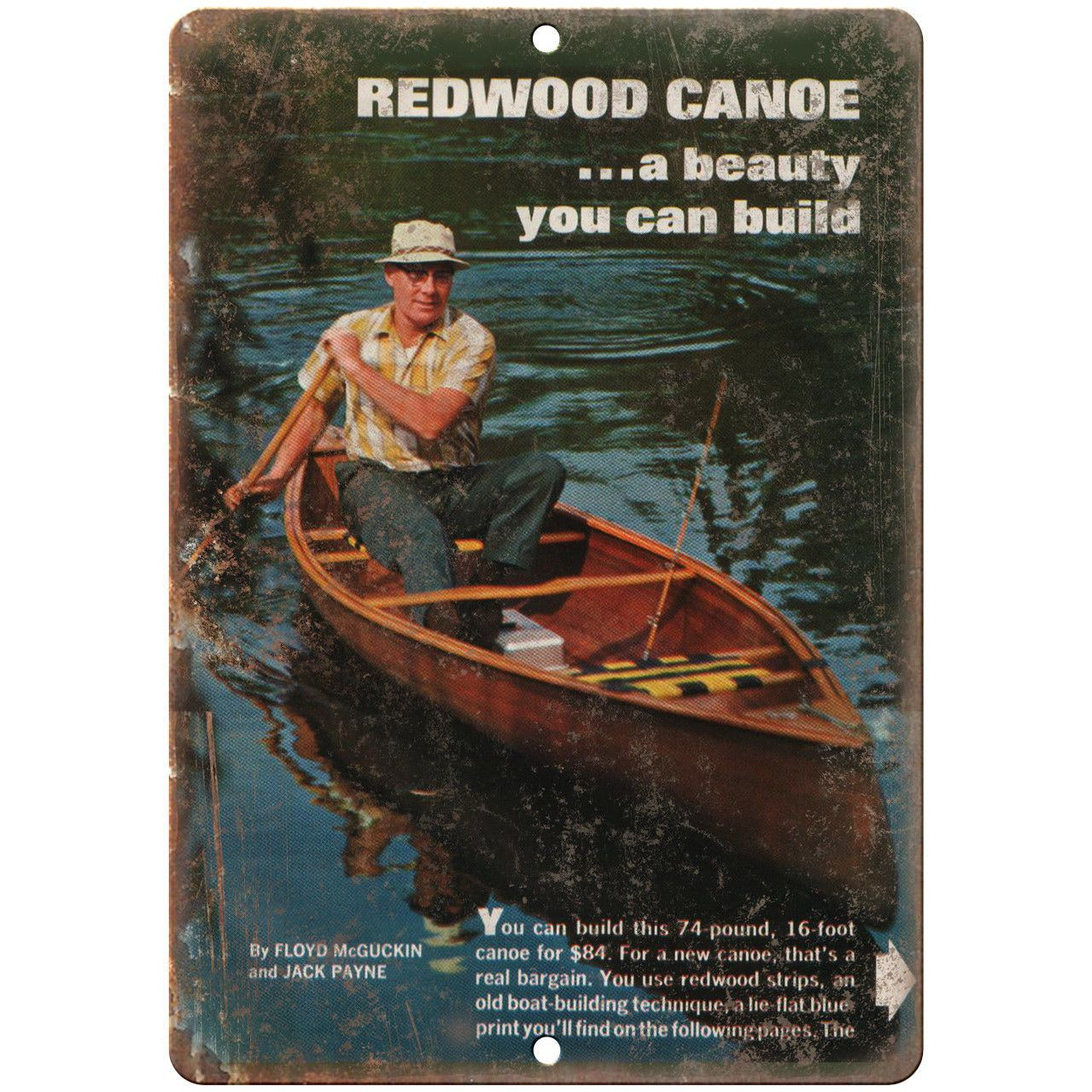The image depicts a worn and vintage sign or booklet cover that features a man in a canoe on still water, possibly a lake. The caption reads, "Redwood Canoe... A Beauty You Can Build" by Floyd McGuckin and Jack Payne. The image showcases a man of European descent with wire-rim glasses, a fishing hat, a checkered shirt, and jeans, rowing a brown wooden canoe on the right side with a fishing rod and tackle box inside the canoe. The background is brown-hued, giving the image an aged feel. Below the main title, the text highlights that one can build a 74-pound, 16-foot canoe for $84 using Redwood strips, an old boat-building technique. An arrow points to additional blueprints on the following pages, indicating instructions to continue. The edges of the image are worn, with white wear spots, and it has holes at the top and bottom, suggesting it was once nailed to a surface.